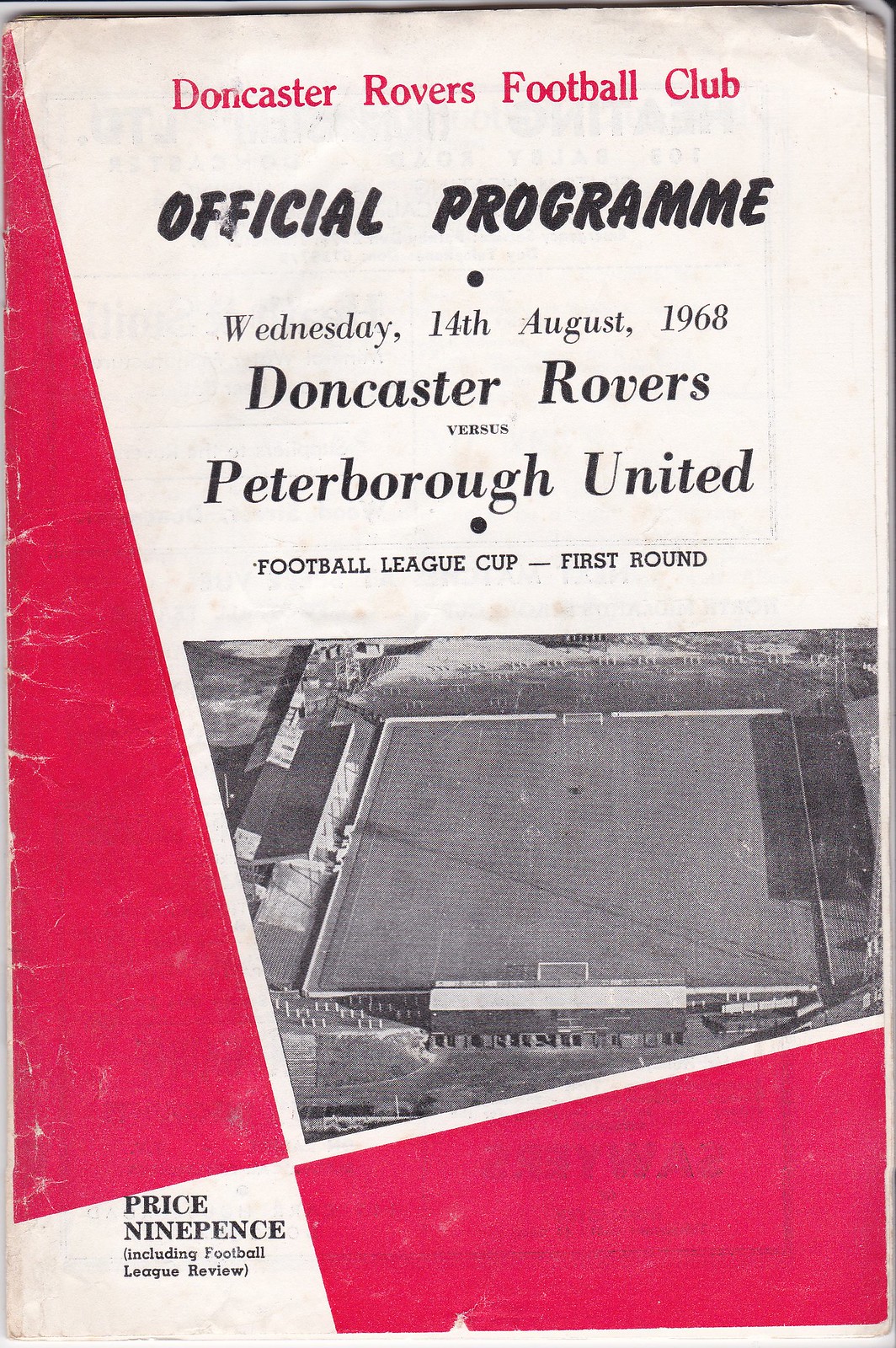This image depicts the cover of an official football program for a match between Doncaster Rovers and Peterborough United, played on Wednesday, August 14th, 1968, in the first round of the Football League Cup. The cover predominantly features a red and white color scheme, with red text at the top reading "Doncaster Rovers Football Club" against a white background. Below this, in black text, are the details, "Official Program Wednesday, 14th August 1968 Doncaster Rovers versus Peterborough United Football League Cup First Round."

The center of the cover showcases a black and white overhead photograph of a soccer stadium where the game took place. Adding a splash of color and personality to the design, red triangles are situated below the photograph, leading to a partially visible next page advertisement in the red area beneath. In the bottom left corner, against a white background, the price is listed in black text as "Price Nine Pence, including Football League Review." There is also a faint, illegible blue stamp on the bottom right, hinting at the program's age and wear. The program is worn, printed on paper, and the top area shows signs of fading.